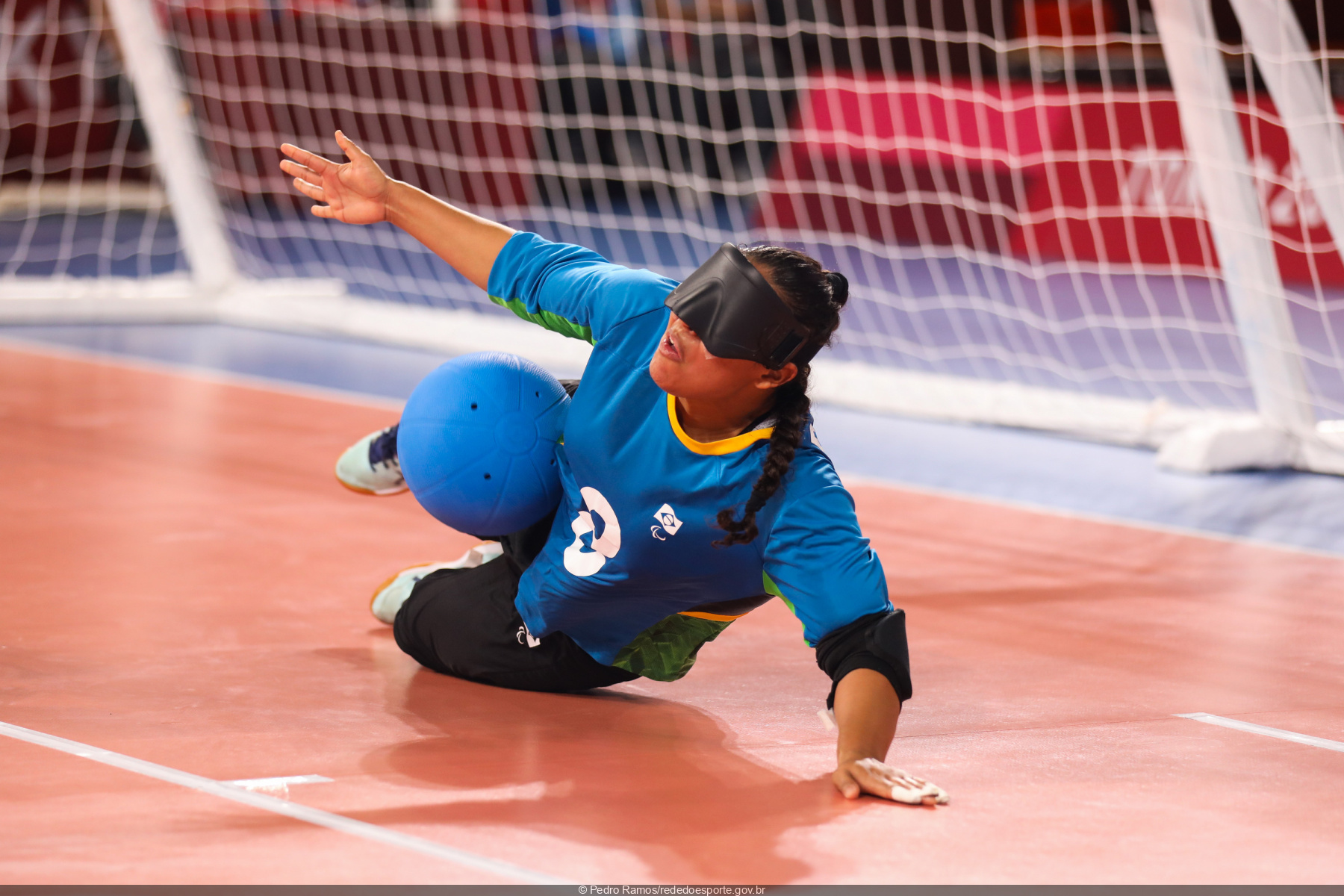In this detailed image, a female athlete, who appears to be either African-American or Southeast Indian, is captured in action on an indoor sports court. She is playing the role of a goalie, visibly engaged in a dynamic moment where she stops a blue ball between her legs while partially lying on the floor. Her long black braid cascades down her back, and she sports a large black blindfold, which might be a thick plastic mask, covering her eyes suggesting a unique or adapted version of a sport, possibly involving virtual reality elements. She wears a long-sleeve blue shirt featuring an orange collar, paired with black pants and white sneakers. Additionally, an elbow pad can be seen on her left elbow. The court underneath her is a reddish wooden floor marked with white lines, leading up to a large, white goalpost with a white mesh net directly behind her, indicating she is centered in front of the goal area attempting to defend it.